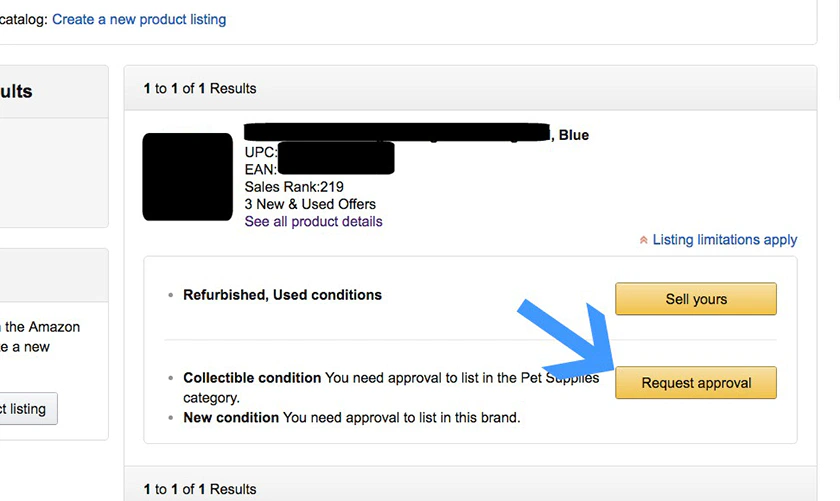**Detailed Caption:**

The image showcases a screenshot of an Amazon product listing page in which a new product is being created. The left section of the screen is partially cut off, displaying limited information about the site. The visible part reads "Amazon," indicating that this listing pertains to their platform. The main focus of the screenshot is centered on the product listing interface, starting with a photo of the item, although much of the critical information has been redacted using a photo editor.

The redacted areas include important product details at the top of the interface. Additionally, a blue arrow, likely added through a photo editor, points towards the orange "Request Approval" button on the right-hand side. Directly above this button is another labeled "Sell Yours," suggesting options available for listing the product for sale.

Further down the page, the text mentions a sales rank of 219 and shows options for "three new and used offers," along with a link to view all products in "refurbished conditions" and the "sell yours" option under the "collectible condition" section. The text indicates users need approval to list items in the "pet supplies" category or under certain brands, highlighted by a red upward-pointing arrow with the note "listing limitations apply."

This screenshot captures the essence of the Amazon product listing approval process, showing the sections where potential sellers are prompted to seek approval for their listings. The snapshot ends with the repeating indication of "one to one of one results," and a final note in blue text, although partially blocked, suggesting more information that is hidden.